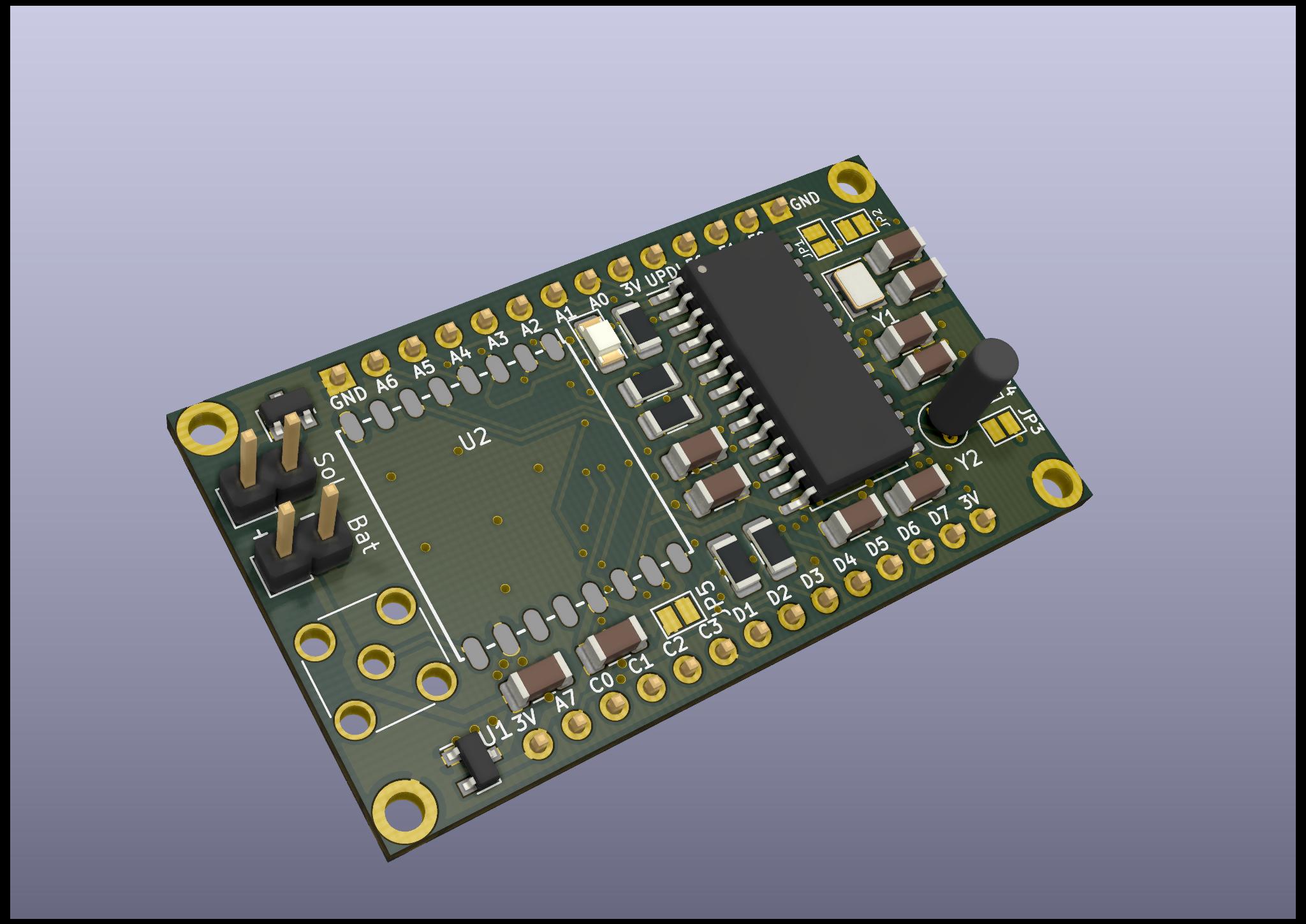The image features a computerized digital illustration of a green circuit board adorned with numerous intricate details. The board exhibits several small gold-bordered punch-out holes and various components, including black and brown rectangular capacitors. A notably large black component occupies the upper right corner, held in place with silver-like pins. The circuit board is marked with several labels, such as "SOL," "BAT," "GND," and "Y1," and features rows of yellow notches labeled with "3V," "A7," "C0," "C1," "C2," "C3," "D1" to "D7," "Y2," "U1," and "U2." The background transitions from a light gray at the bottom to an almost white at the top, framed by a thin black border, and possibly gives off a lilac or purple-gray hue. The detailed layout and nomenclature suggest it is a representation of an electronic control or circuit board typically found within electrical devices.